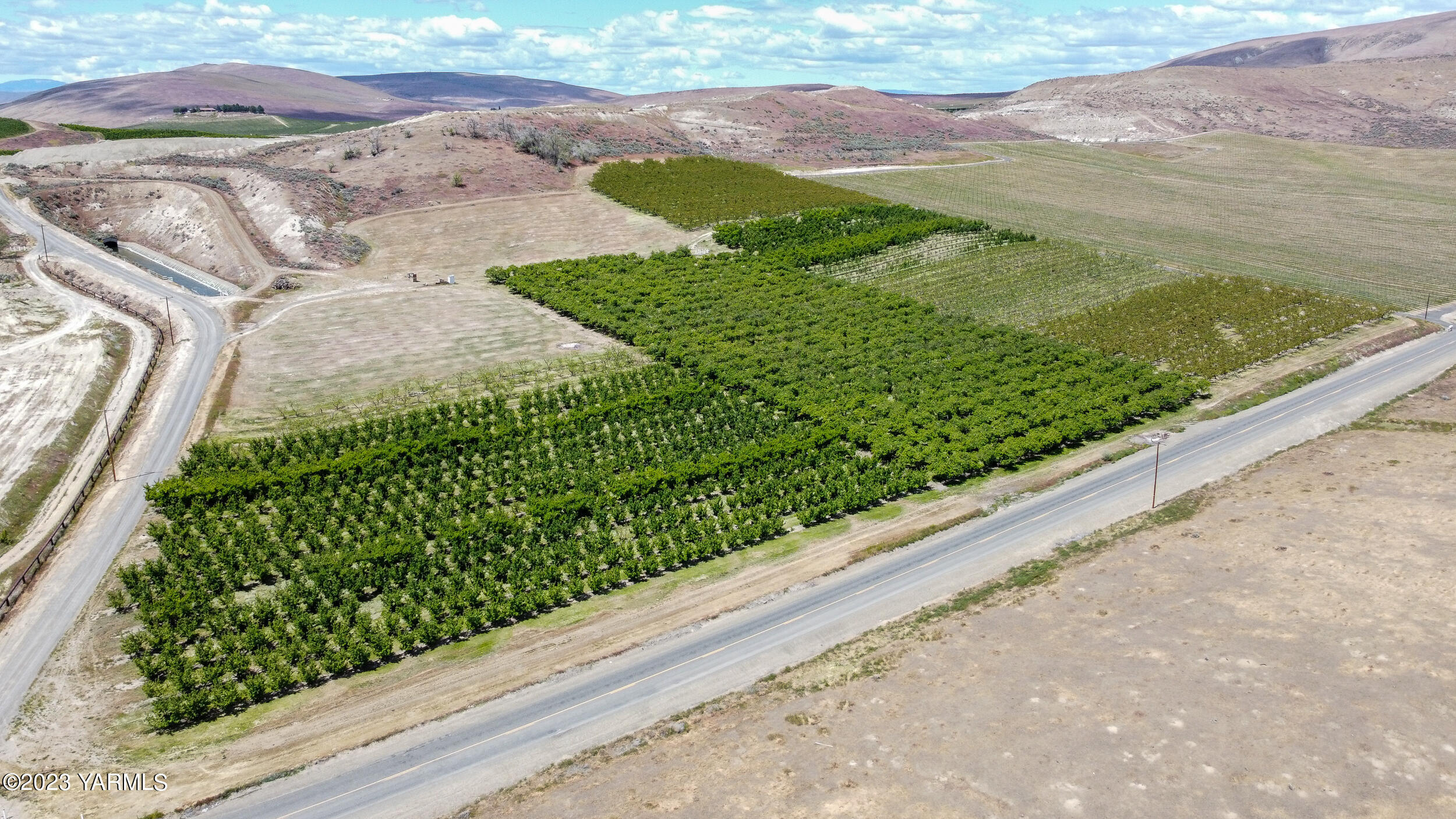This aerial photograph, likely taken by a drone or helicopter, vividly showcases a distinct farmland set against an arid, desert-like backdrop. The focal point of the image is a vast expanse of cultivated land, predominantly featuring two rectangular plots densely populated with uniformly aligned bushes of a vibrant green hue. These central plots suggest the meticulous planning often associated with vineyards, although the exact crop remains unidentified.

To the left and lower left of the middle rectangular field, there are additional rectangular patches hosting shorter, lighter green plants, indicating crops at different growth stages or of different varieties. The farmland is meticulously organized into rows and squares, creating a striking contrast with the surrounding barren terrain.

Encircling these fertile plots are several stark, yellow-lined roads, one extending from the bottom left corner towards the middle right, and another branching off to the left side of the image. These roads are accompanied by light poles and guardrails, highlighting the infrastructure within the otherwise desolate area. The landscape transitions from the cultivated green fields to expansive stretches of brown, sandy soil, giving a sense of an oasis amid a desert.

In the background, a series of modestly sized, brown hills rise under a hazy blue sky dotted with clouds, adding depth to the scene while underscoring the arid conditions dominating the periphery of this lush, green farmland.